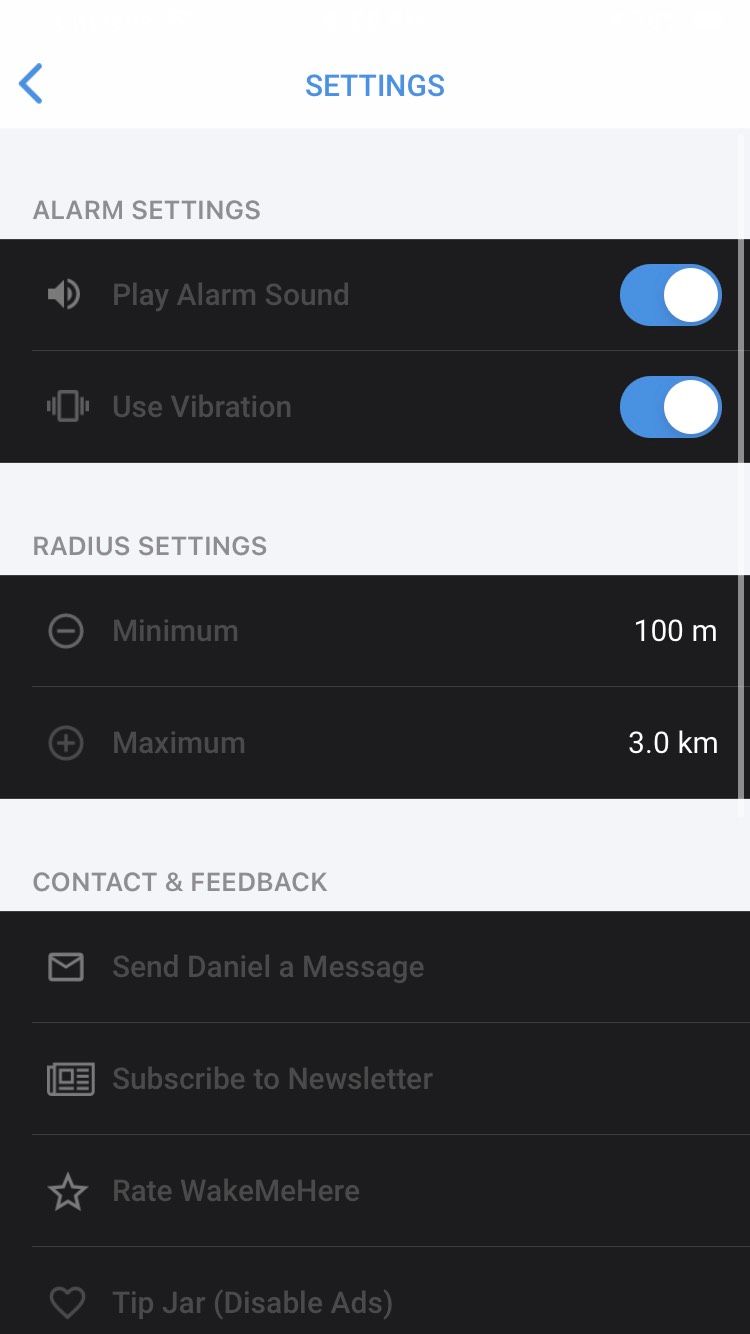The image illustrates an interface with a predominantly blue background at the top. Within this blue section, there are icons including a left arrow and a settings symbol, both in blue. Below this, the interface transitions to a detailed display of alarm settings within a large black box. This section includes an option labeled "Play Alarm Sound," accompanied by a white circle toggle switch set against a blue backdrop. Additionally, there's a "Use Vibrations" option that also features a similar toggle switch design.

Moving further down, the interface showcases "Radius Settings," again within a large black box. This section provides options to "Minimize," with a value stated as "100 M" on the right side, and "Maximize," with a corresponding value of "3.0 KM."

The bottom portion of the interface returns to a blue background and includes sections for "Contact and Feedback," featuring options like "Send Daniel a Message," "Subscribe to Newsletter," "Rate Wake Me Here," "Tip Jar," and "Disable Ads," each within individual large black boxes.